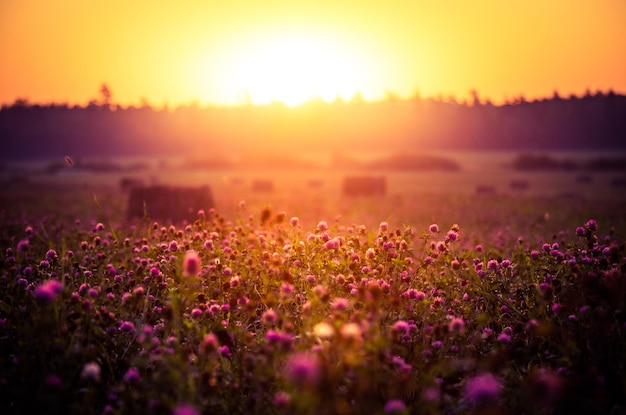The image depicts a warm-toned photograph of a serene outdoor field at either sunrise or sunset. The foreground is alive with an array of wildflowers, predominantly small purple and pink blooms, interspersed with some lighter yellow ones. The grass in this area is short, allowing the vibrant flowers to stand out. Towards the middle of the image, there are several hay bales scattered randomly across the grassy field, although this section appears slightly faded, making the details less distinct. At the top, a tree line forms a dark silhouette against the bright backdrop of the rising or setting sun. The sky transitions from a brilliant yellow around the sun to deeper shades of orange toward the edges, casting a glowing effect that bathes the entire scene in a warm, inviting light. The very bottom corners of the image are darker, adding depth and framing the colorful foreground with wildflowers.